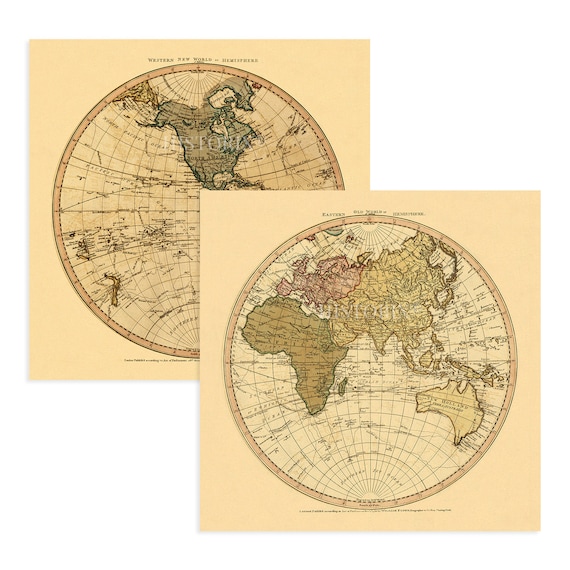This detailed photograph features two overlapping, vintage-looking diagrams of flattened globes, reminiscent of antique maps on aged, off-white, cream-colored paper. The top image, closer to the viewer, displays the continents of Africa, Europe, Asia, and Australia, depicted in subtle, earthy tones like greenish-yellow, pinkish-red, and light yellow for distinct regions. Visible in this image are the detailed lines of longitude and latitude, further emphasizing its old-world charm. The background picture portrays a similar ancient map theme, predominantly showcasing North America in light-blue hues, with possible hints of South America slightly obscured by the top image, and bits of the Pacific Islands. Both maps feature country names, bodies of water, and various other geographical details, adding depth to the historical cartographic presentation. At the top of the images is a faint, partially legible title that appears to read "Webster's New World Ephemeris," enhancing the nostalgic, scholarly aesthetic of the photograph.